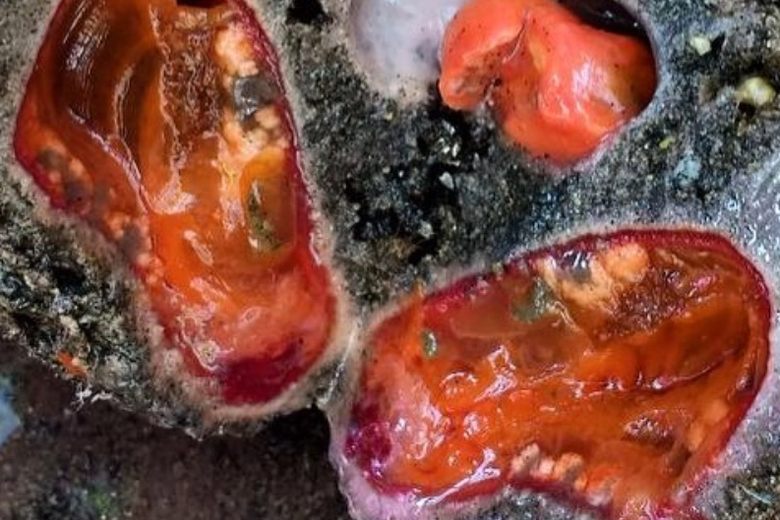The color photograph, presented in a wide vertical rectangular format, captures a close-up view of what appears to be a cooking process. The backdrop is a gradient of dark gray to black, enhancing the vivid colors in the foreground. Three red blobs, possibly resembling tomatoes or pieces of meat, are positioned in a bubbling clear liquid. The liquid is frothy with white bubbles, indicating that it is likely hot and cooking. The largest blob, situated on the left, has a somewhat rectangular shape with a curved edge and displays hints of black within its semi-translucent red surface. Another similarly sized blob is located below and to the right. The smallest blob, positioned above, is a lighter shade of red and lies next to a small white blob. Two of the red blobs are garnished with green specks and some white, adding texture and contrast to the image. The overall smooth surfaces and the bubbling liquid suggest that these blobs may indeed be meat cooking in oil.